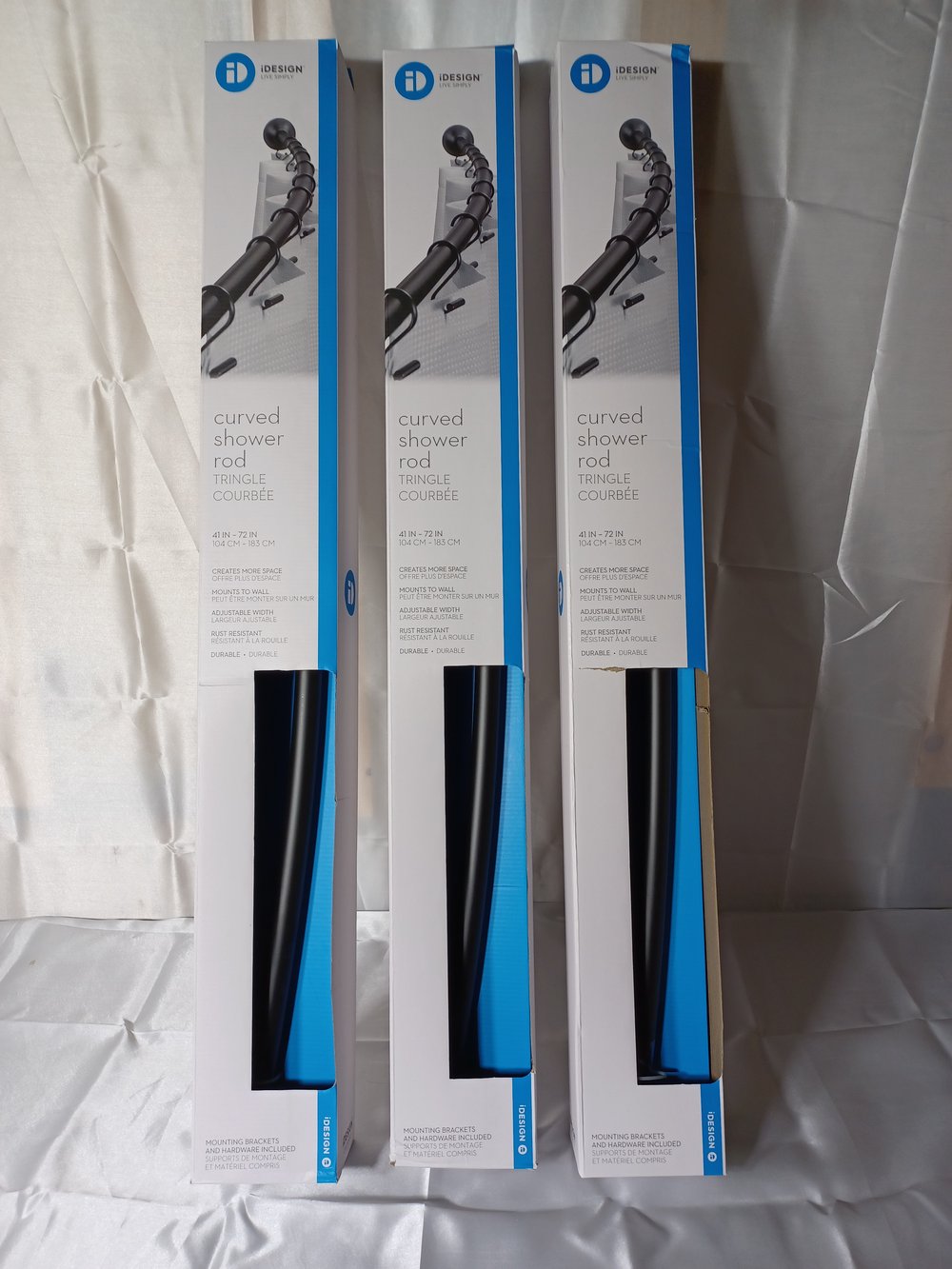In the image, taken indoors, three identical, narrow, rectangular boxes containing black curved shower rods are neatly lined up, leaning against a white wall that meets a white floor. The white background appears to be a satin-like fabric curtain, recently unfolded as evidenced by the numerous square creases throughout. Each box is approximately four inches high and half an inch wide. The upper section of the boxes features a blue circle with white letters "ID," and to the right of this, in gray text, the brand name "I-design" is displayed. Below this, a descriptive picture and text about the curved black shower rods is provided. The lower part of each box includes a clear cutout, allowing the actual black cylindrical rods to be visible. Along the right side of the boxes runs a vertical blue stripe, complementing the blue circle on the upper left. The scene creates a composed and detailed presentation of the shower rod products against the textured white curtain backdrop.